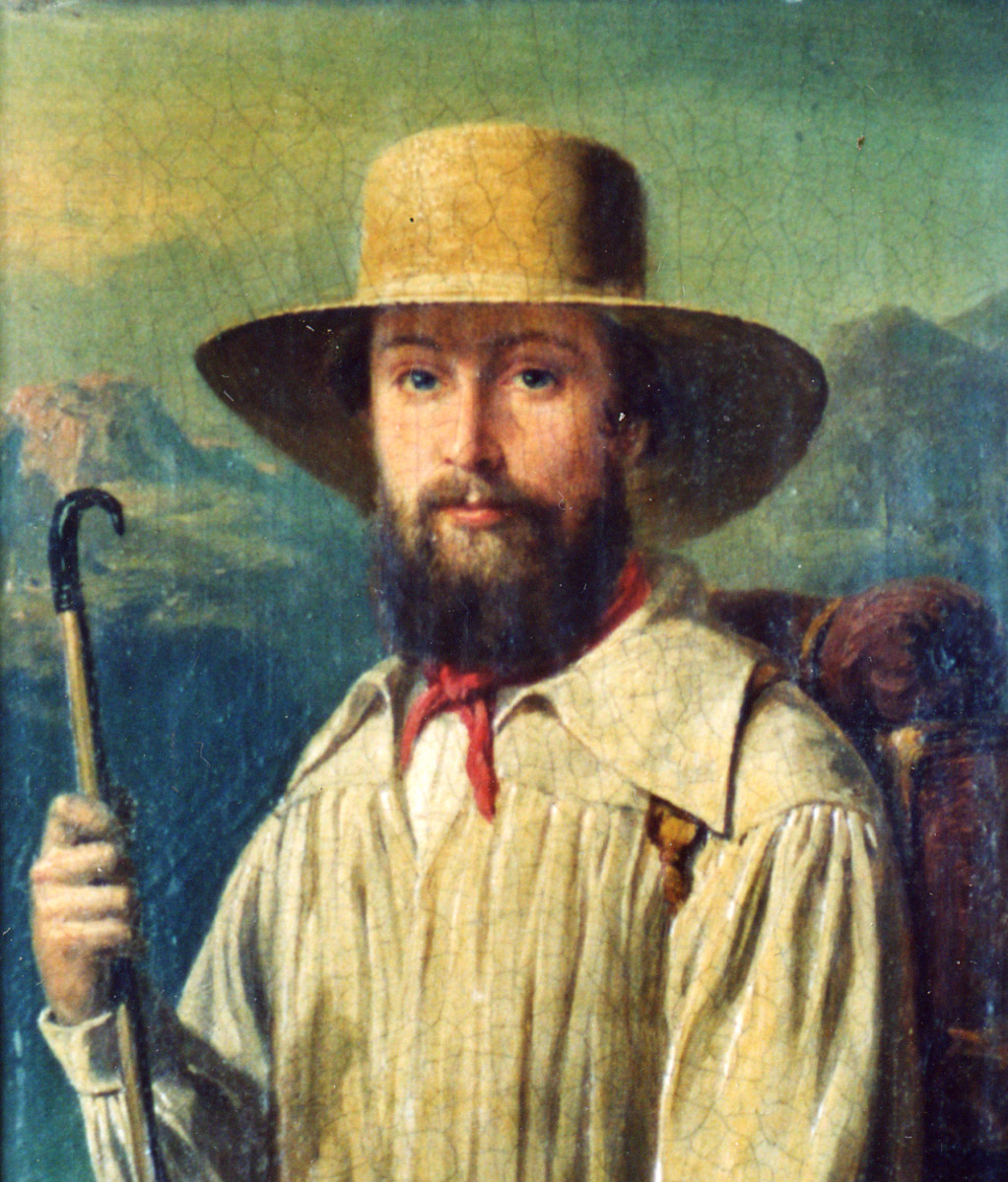This photograph captures a timeworn painting, showcasing the rich textures and history evident in its cracked and weathered surface. The portrait features a bearded man clad in vintage hiking attire, who stands resolutely against a backdrop of towering, rugged mountains. His ensemble includes a brown sun hat, a red kerchief elegantly tied around his neck, and a sturdy backpack strapped to his shoulders. In his hand, he grips a long, well-worn cane, suggesting many years of arduous treks. The detailed mountain range on either side of the man, along with the serene blue sky in the background, enhances the sense of adventure and timelessness encapsulated in this evocative artwork.